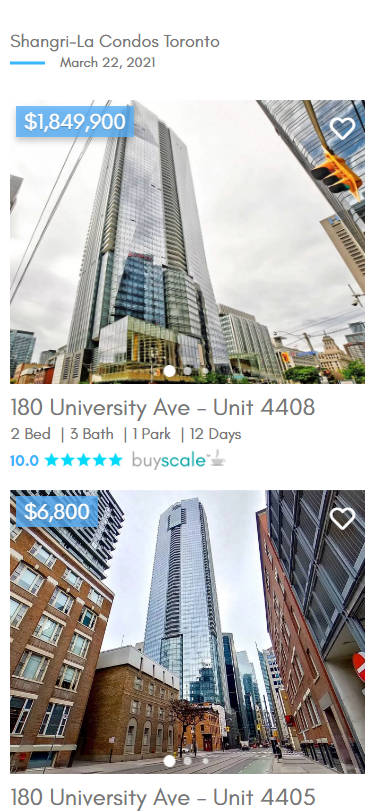**Descriptive Caption:**

The image features two property listings, both in Toronto. 

**Top Listing:**
- **Title:** Shangri-La Candles Toronto
- **Date:** March 22, 2021
- **Price:** $1,849,900 (Display: white text on a blue background)
- **Image:** A tall building under a grey, cloudy sky.
- **Details:** 
  - Address: Arlington 80, Universities Avenue, Unit 4408
  - Features: 2 beds, 3 baths, 1 parking spot; listed for 12 days
  - Rating: 5 stars (blue stars)
  - Notations: 'Scale' written in blue; overall text in black

**Bottom Listing:**
- **Price:** $6,800
- **Image:** A building surrounded by other brown buildings.
- **Details:**
  - Address: 180 Universities Avenue, Unit 405

This detailed description provides a clear and organized visualization of the properties and their specifics.